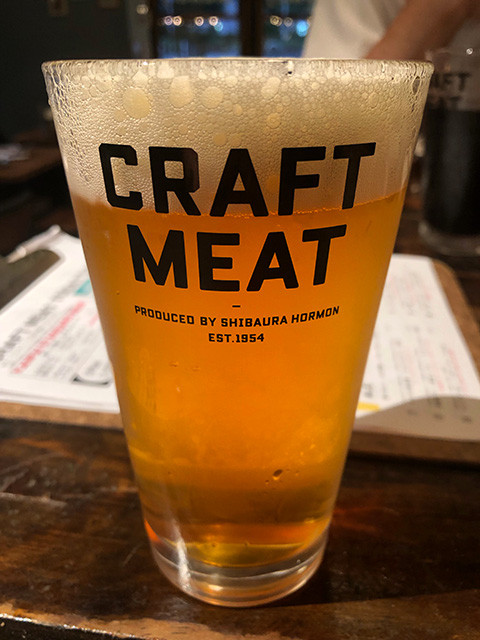A clear pint glass of golden, foam-capped beer, labeled prominently with "Craft Meat" in bold black letters, and “Produced by Shibaura Horman, Est. 1954” beneath, rests on a wooden bar surface. The image foregrounds this glass, nearly occupying the entire frame. Behind it lies an open clipboard with indistinguishable writing. Further back, a person in a white shirt, right arm raised, and holding a similar glass, is seen. The setting seems to be a bar, with doors or windows faintly visible in the backdrop.